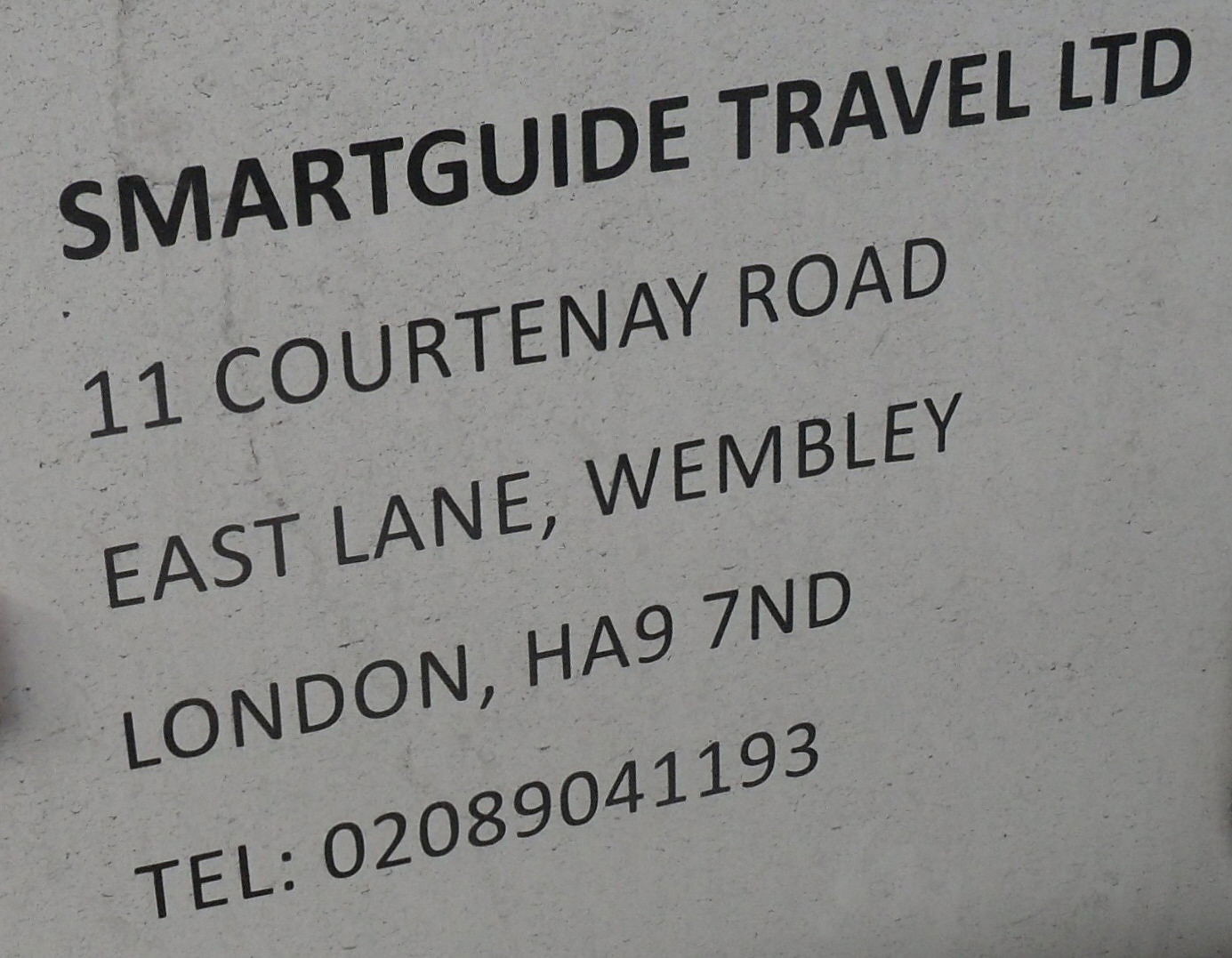The photograph depicts a simple black and white sign with bold black text on a white background. At the top, in dark black, bold letters, it says "SmartGuide Travel Limited, LTD." Below that, in slightly smaller, but still prominent font, the address is listed: "11 Courtenay Road, East Lane, Wembley, London, HA97ND." At the bottom, also in black letters, it reads "TEL: 0208-904-1193." The text appears slightly off-kilter, suggesting that the photograph was taken at an angle. The sign may be an engraving on a cement wall or printed on light gray paper, giving the letters a very dark gray to black appearance.